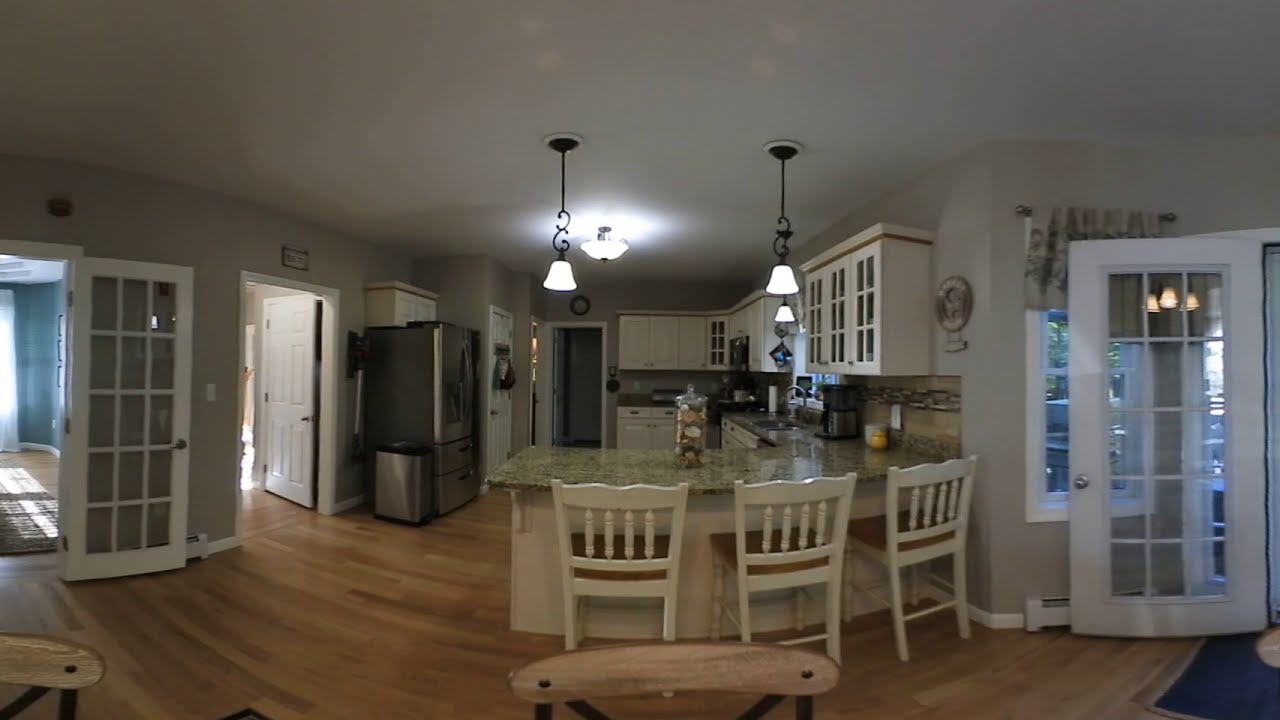The image depicts a cozy, country chic kitchen with a slight panoramic distortion. At the forefront, three whitewashed bar chairs line a small counter with a glossy green and black granite surface, underpinned by an off-white cream base. The wooden floor is adorned with polished planks. On the right, the kitchen features a large stainless steel refrigerator flanked by a closed door with something hanging on it and an open door revealing a sunlit room with light blue walls. Additional light floods in from another open paneled door revealing lush green vegetation outside.

The back wall hosts a series of cabinets: those on the right have glass windows, while the far end houses three solid door cabinets. A mix of decorative ceiling lights includes a central round light and three hanging lamps with white bulbs. The overall color scheme includes whitewashed cabinetry and grayish-white walls, creating a welcoming, backcountry aesthetic. Sunlight streams in, contributing to the warmth and charm of this beautifully maintained home.